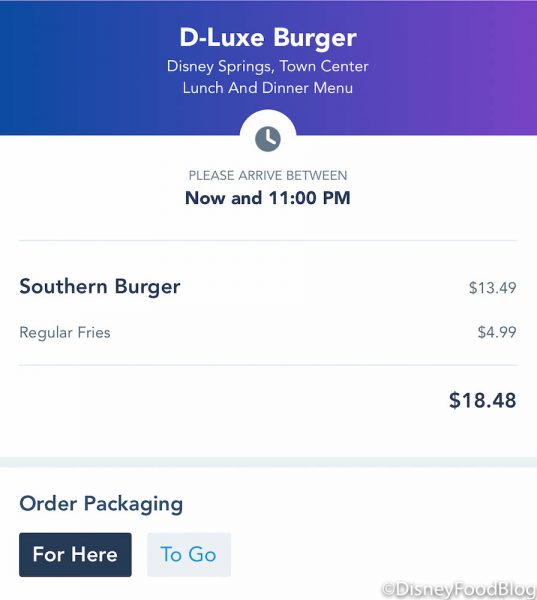A user is in the process of ordering food online from D-Luxe Burger at Disney Springs, Town Center. The interface features a gradient bar at the top that transitions from blue on the left to purple on the right. The text on the bar states "D-Luxe Burger Disney Springs, Town Center," indicating that lunch and dinner menus are available. The user is prompted to arrive between now and 11 p.m., with a small clock icon situated above this notification.

They are ordering a Southern Burger priced at $13.49, and regular fries for $4.99, bringing the total to $18.48. Options for order packaging are provided as "For Here" or "To Go," with "For Here" highlighted in blue with white text, and "To Go" shown in gray with turquoise font. The bottom right corner features a "Copyright Disney Food Blog" watermark in white text with a gray drop shadow.

The color scheme includes blue, purple, gray, black, white, and turquoise on a white background. The interface’s combination of these colors provides a visually appealing and user-friendly experience, though the price may seem high, it aligns with typical Disneyland pricing.